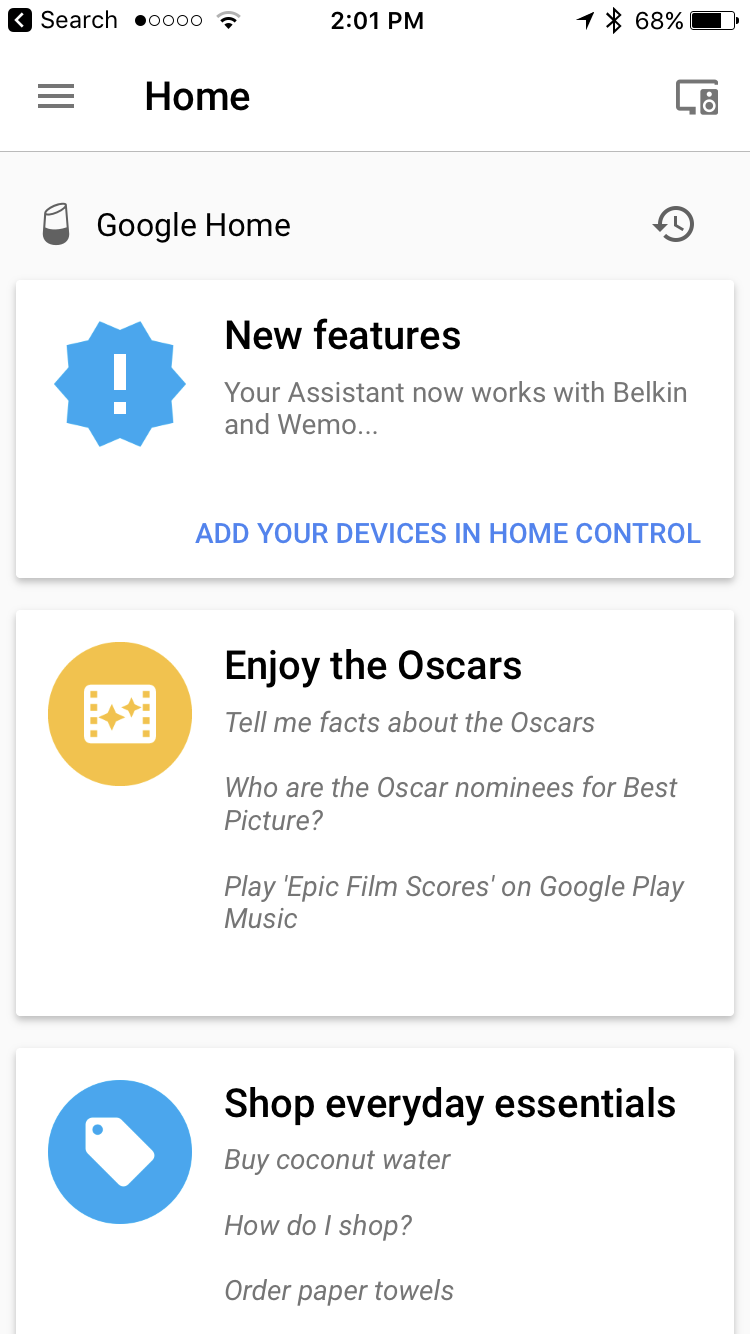The image features a digital interface with various elements, starting from the top-left corner:

- A black square with a left-pointing arrow and the label "Search" adjacent to it.
- A black circle appears next, followed by four circles outlined in grey.
- A Wi-Fi symbol is displayed, along with the time "2:01 PM."

On the top-right corner are:
- An icon resembling a paper airplane.
- A Bluetooth symbol.
- A number "68%" indicating a level, likely battery percentage.
- A battery icon.

Moving back to the left-hand side, beneath the time display:
- Three stacked lines, commonly referred to as a “hamburger” menu, with the label "Home" in black font.

Directly under these elements are a series of shapes:
- A form resembling part of a rectangle.
- A small grey rectangle featuring a white dot and an outlined white circle.

A grey line runs beneath these shapes, followed by:
- A light grey rectangle.

The central part of the interface includes:
- A graphic of a tilted, black-bottomed, white-topped cup-like shape with the label "Google Home."
- A circular icon with an arrow and clock arms inside it.
- A white rectangle containing a starburst icon with an exclamation point. The starburst is blue, the exclamation point is white, and the text reads: "New features: Your Assistant now works with Belkin and Wemo…"
- A blue line with the text: "Add your devices in Home Control."

Further down, within another white rectangle:
- A blue circle featuring a white rectangle adorned with stars and dots.
- Text promoting the Oscars: "Enjoy the Oscars - Tell me facts about the Oscars, Who are the Oscar nominees for Best Picture, Play epic film scores on Google Play Music."

At the bottom of the interface, partially visible, there's:
- Another white rectangle with a blue circle containing a tag. The tag has the label: "Shop everyday essentials: Buy coconut water, How do I shop?, Order paper towels."

This detailed composition provides a clear and structured view of the digital interface's various interactive and informational elements.